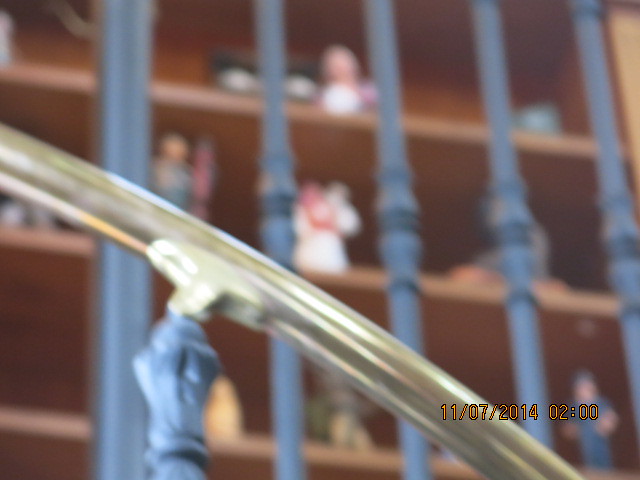This photograph captures a beautifully ornate staircase railing, adorned with a warm golden-bronze hue. The artistic craftsmanship is evident in the detailed design of the railing, which elegantly sweeps upward. A central post anchors the railing as it ascends diagonally before transitioning into a vertical section. In the background, the staircase railing intersects with a cabinet or set of shelves. These shelves are tastefully decorated with various figurines, adding a charming and intricate backdrop to the sophisticated staircase feature.